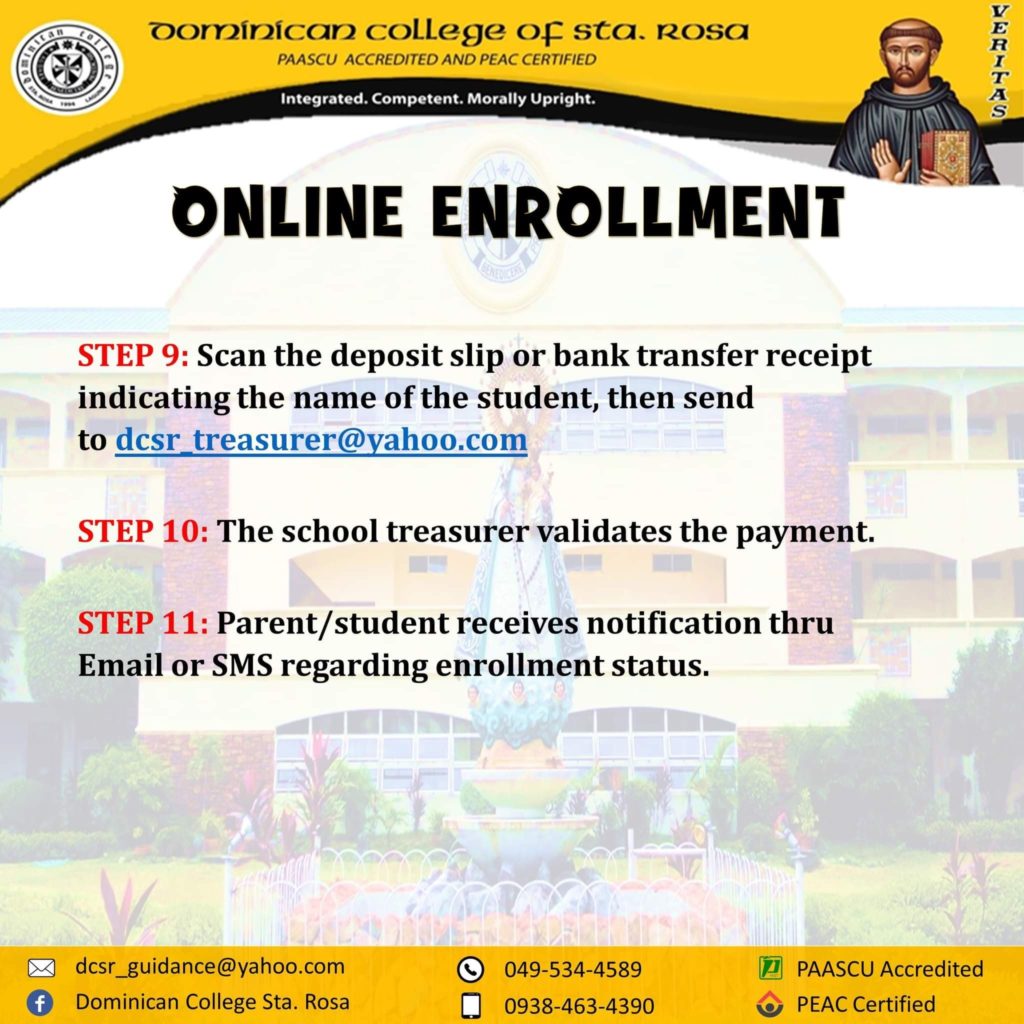This is a detailed and cleaned-up caption for the described image:

---

Webpage for the Dominican College of Santa Rosa's Online Enrollment (Steps 9-11):

The webpage features a distinctive yellow bar at the top with a wavy bottom edge. In the upper left corner, a black and white logo of the Dominican College of Santa Rosa is prominently displayed. On the right side, an image of what appears to be an apostle or saint is present, accompanied by the word "Veritas" written vertically next to it.

At the very top center of the page, "Dominican College of Santa Rosa, PAASCU Accredited and PEAC Certified" is written in black text. Directly below, within the wavy black section, the phrase "Integrated Component Morally Upright" is inscribed.

The main header below this section reads "ONLINE ENROLLMENT" in large uppercase black font. The enrollment instructions are laid out as follows:

- **Step 9:** (in red text) "Scan the deposit slip or bank transfer receipt indicating the name of the student, then send to [website/email address]." (written in black text)
- **Step 10:** (in red text) "The school treasurer validates the payment." (written in black text)
- **Step 11:** (in red text) "Parent/student receives notification through email or SMS regarding enrollment status." (written in black text)

Overall, the page provides clear and structured guidance for the enrollment process.